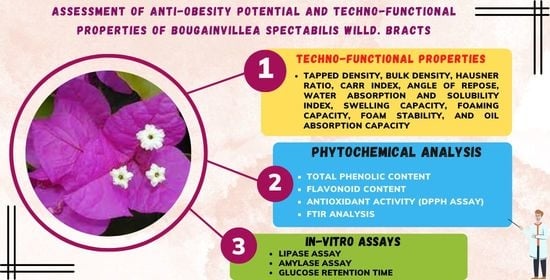The poster is a detailed infographic predominantly light pink in color, dedicated to the "Assessment of Anti-Obesity Potential and Techno-Functional Properties of Bougainvillea spectabilis Wild Bracts." At the top center of the poster, the title is clearly visible. The central image of the infographic features a circle enclosing a vibrant, purple Bougainvillea spectabilis flower with small white flowers, resembling large, purple leaves.

Surrounding the central image are three bullet points, each in different colors, extending outward from the circle. These points highlight key aspects of the research:

1. **Techno-Functional Properties**: This section lists several detailed properties including tapped density, bulk density, Hausner ratio, Carr index, angle of repose, water absorption, solubility index, swelling capacity, foaming capacity, foam stability, and oil absorption capacity.

2. **Phytochemical Analysis**: Detailed parameters here include total phenolic content, flavonoid content, antioxidant activity (measured by DPPH assay), and FTIR analysis.

3. **In vitro Assays**: This final section outlines various assays such as lipase assay, amylase assay, and glucose retention time.

At the bottom of the poster, a man in a white lab coat with dark pants stands upright, adding a professional and personal touch to the presentation.